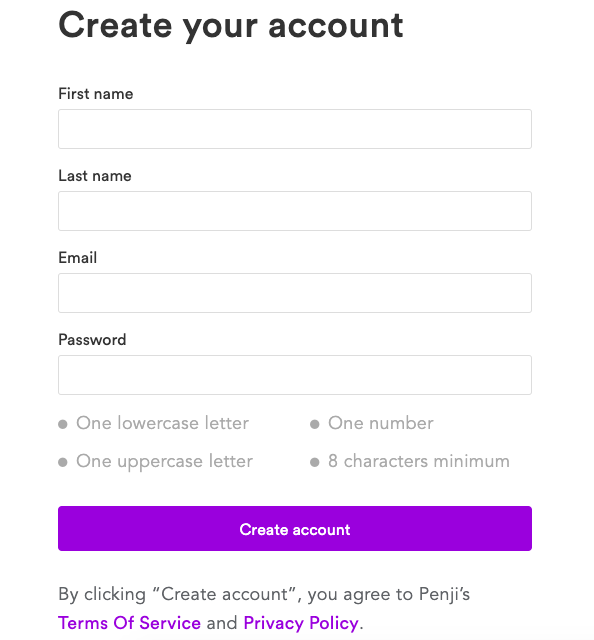The image depicts a user registration page, prominently featuring the title "Create Your Account" in bold black letters at the top. The form starts with a text box for the user's first name, followed by another for the last name. Below these, there is a text box for entering an email address, and beneath that, a password text box. Guidelines for the password are listed underneath: it must include at least one lowercase letter, one uppercase letter, one number, and be a minimum of 8 characters long. Further down, a wide, purple bar labeled "CREATE ACCOUNT" spans the width of the page. Below this bar, there's a notice stating, "By clicking 'CREATE ACCOUNT', you agree to PENG's Terms of Service and Privacy Policy," with both terms highlighted in purple. The background of the entire page is white, except for the purple highlights and button.